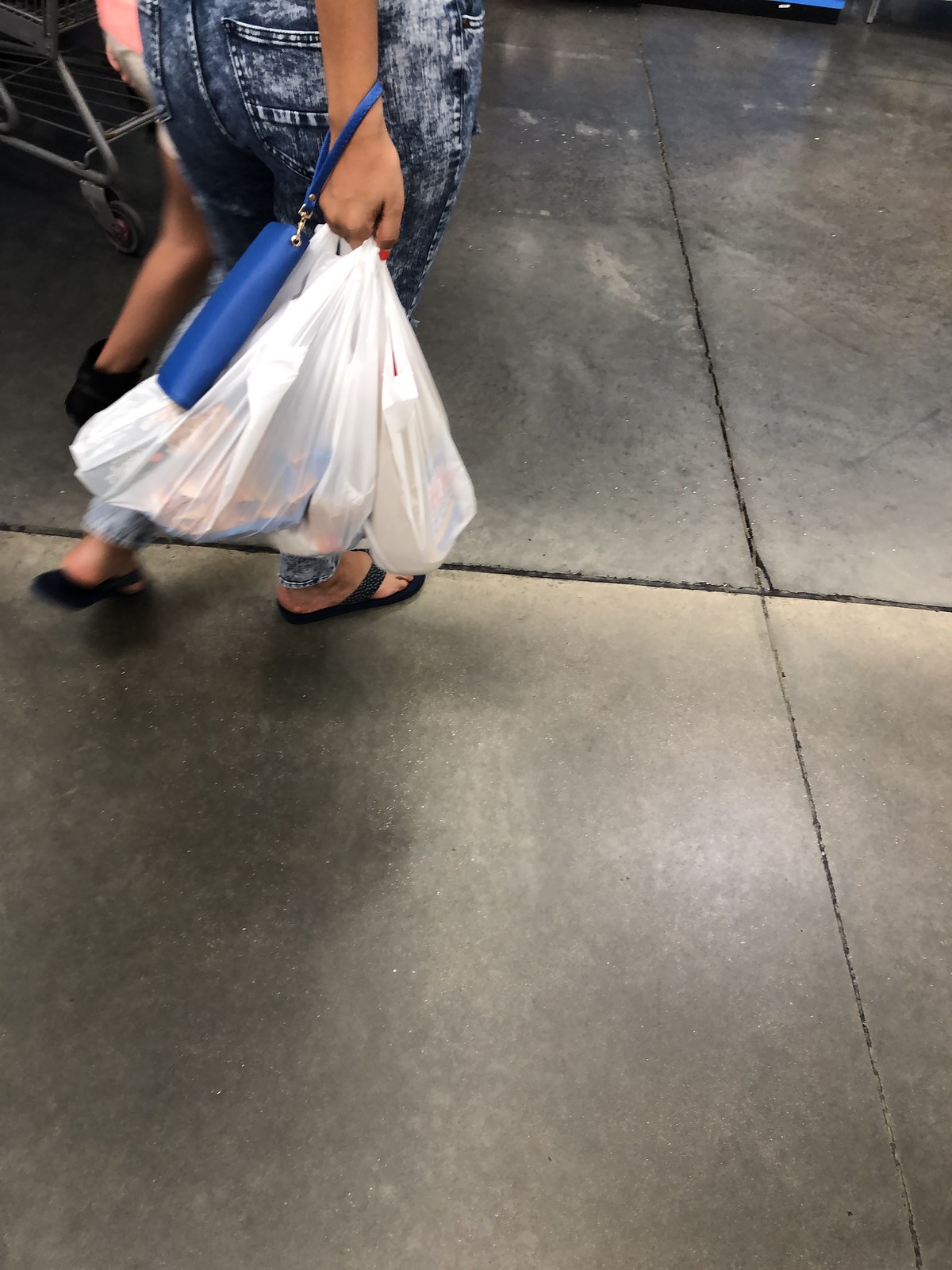The photograph captures a downward view of a shiny, gray, and light-brown tiled floor, likely in a grocery store. The large, square concrete tiles feature deep black joints, with the intersections forming a notable point towards the right of the image. The tiles are intersected by lines running horizontally across the middle and diagonally from the bottom right corner up toward the left. In the upper left corner, a grocery cart wheel is visible. In the background, a woman’s legs are seen from the waist down. She wears tie-dye style dark blue jeans with white accents around the hip, black strapped sandals, and carries several white, slightly translucent grocery bags revealing patches of blue and yellow inside. A blue wristlet purse hangs from her wrist, resting on the bags. Accompanying her is another person, partially visible, donning a pink blouse and walking beside her. The scene suggests they're headed out towards a parking lot, hinted at by a sliver of a blue car seen through a distant window.